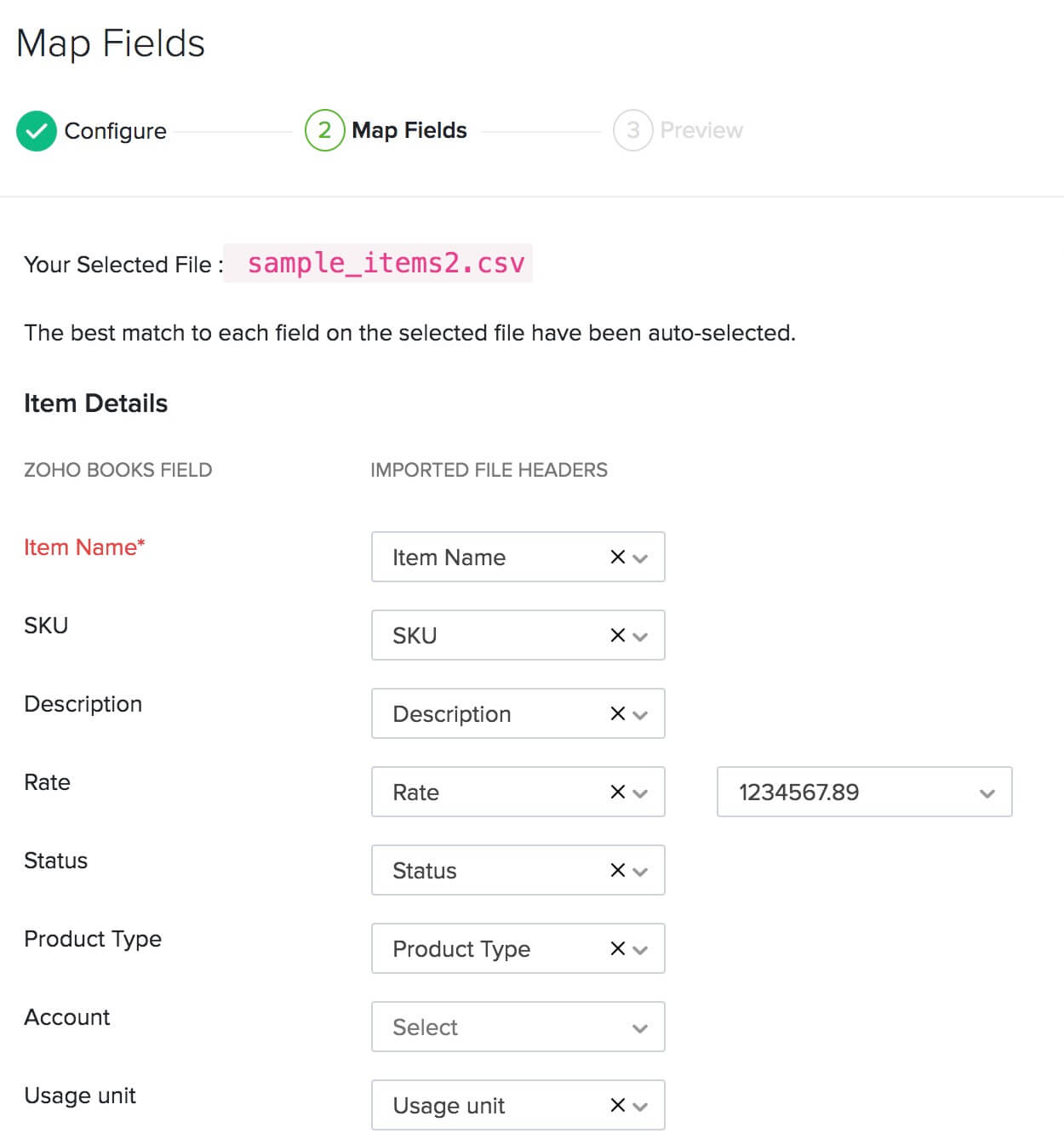The image depicts a multi-step process for configuring document fields in a software interface. At the top, three discrete steps are visually represented: a green checkmark encircled by "1" labeled "Configure," followed by a circled "2" labeled "Map Fields," and a circled "3" labeled "Preview," which is currently grayed out. Below this, a gray line separates these steps from a status message in bold pink text that reads, "Your selected file: sample_items2.csv," contrasting with the remainder of the text in black.

Beneath this is a list indicating the best matches for each field in the selected file, which have been auto-selected. The fields include:

1. **Item Details**:
    - **Zoho Books Field**: Matching with **Imported File Headers**
    - **Item Name**: Item Name (denoted with an asterisk *)
    - **SKU**: SKU
    - **Description**: Description
    - **Rate**: Rate (formatted with decimal values 1.2.3.4.5.6.7.8.9)
    - **Status**: Status
    - **Product Type**: Product Type
    - **Account**: (Selectable through a dropdown menu)
    - **Usage Unit**: Usage Unit

These fields are each followed by an adjacent "X" linked to drop-down menus for selection, presumably allowing further customization or correction of the auto-matched entries.